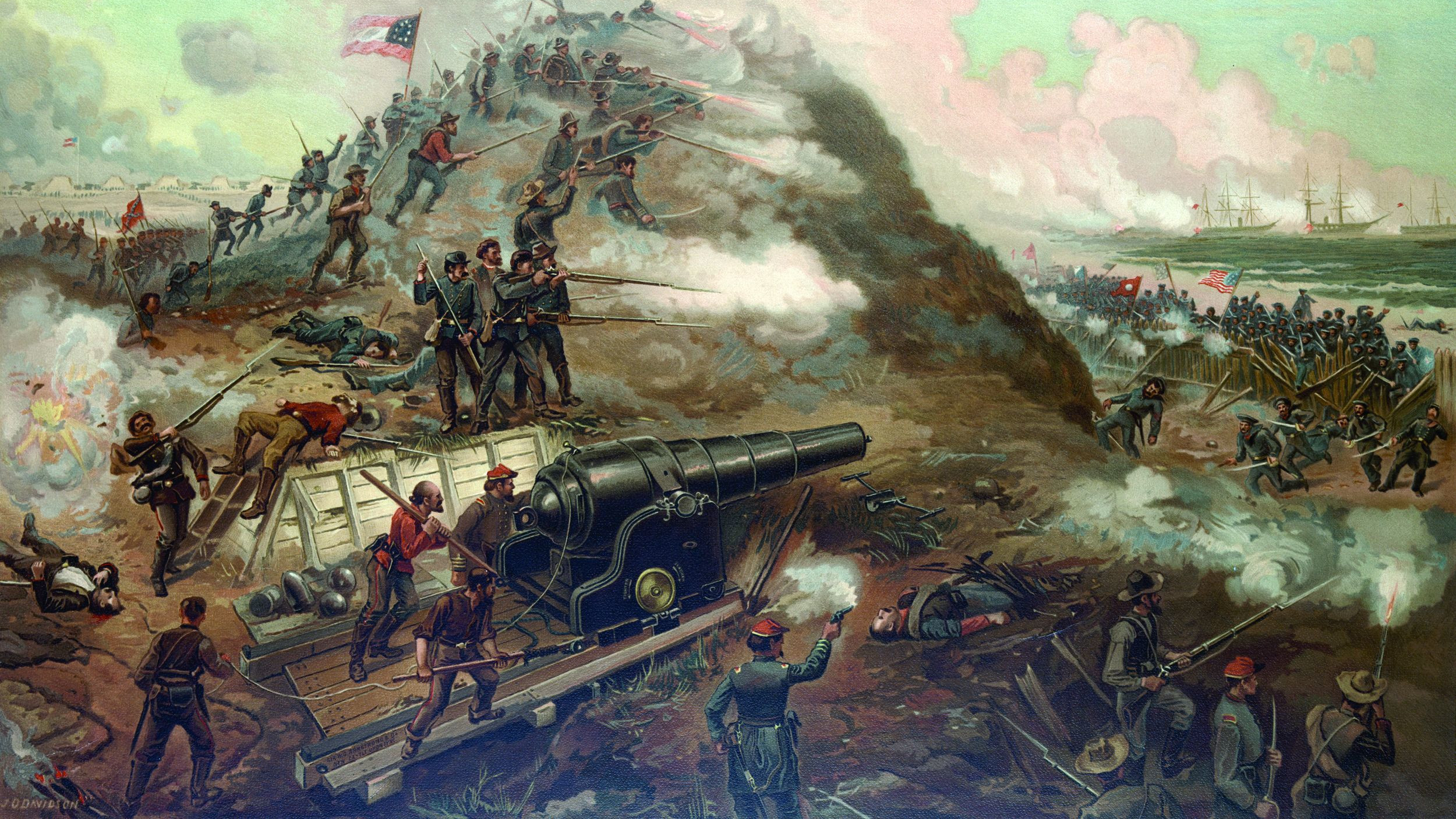This visually intense oil painting captures a dramatic Civil War battlefield teeming with action and chaos. The foreground draws immediate attention to the left, where a group of Confederate soldiers is energetically loading and firing a cannon, enveloping the scene in thick plumes of smoke. Just behind them, a figure prominently hoists the Confederate flag atop a significant hill, asserting the dominance of the Confederate forces in this visual narrative. The battlefield is clouded, not only with the smoke from the cannon fire but also from the musket shots discharged by numerous soldiers attempting to fend off the advancing Union troops. 

On the right-hand side of the image, amidst the frantic blur of battle, Union soldiers, distinguishable by a modern-looking American flag with 13 stars, are valiantly charging through a fence line, swords drawn, trying to break the Confederate barrier. The background, cloaked in smoke and chaos, reveals yet more details; on the top left, hundreds of men are scattered, their presence adding depth and scale. Further in the distance, towards the back of the painting, a few ships are depicted arriving on shore, hinting at reinforcements possibly coming from enemy territory. Every inch of the painting captures the ferocity and tumult of the Civil War, privileging the dramatic prominence and perspective of the Confederate forces while highlighting the relentless charge of the Union Army.